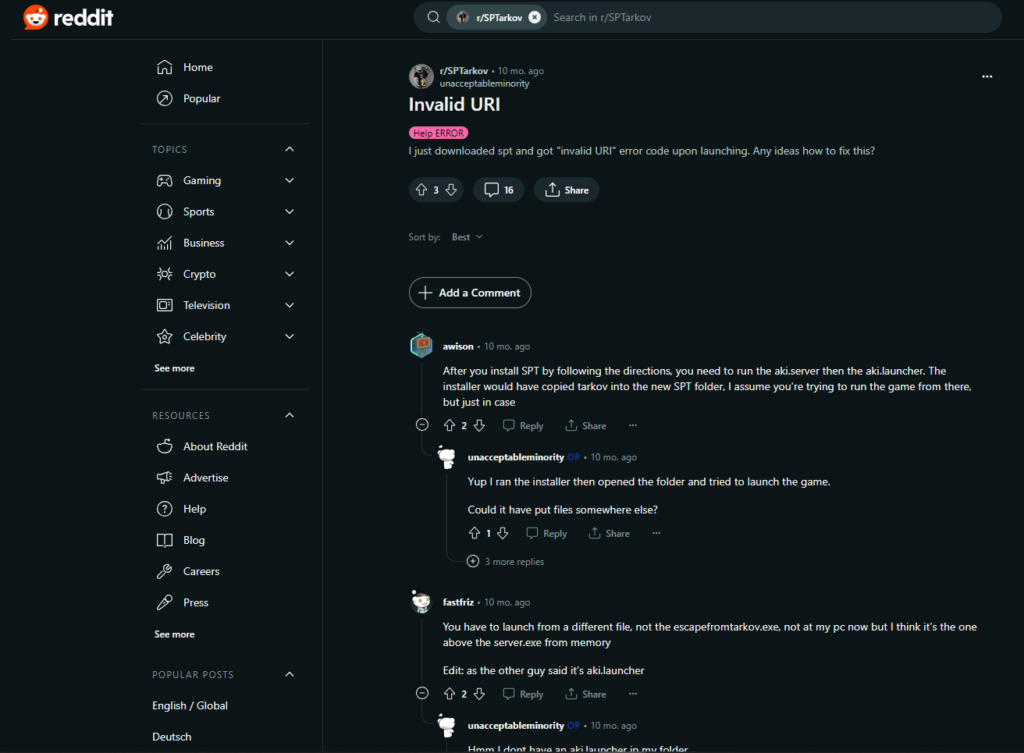In the top left corner of the Reddit website screenshot, the distinctive Reddit logo is prominently displayed — an orange speech bubble with a white alien face inside, sporting a smile. To the right of the logo, there is a search bar followed by a tab labeled "r/SPTarkov". 

On the left side of the page, a navigation bar includes various icons and categories such as Home, Popular, All, Topics, Gaming, Sports, Business, Crypto, Television, Celebrity, and more, each equipped with drop-down menus. Additional links include Resources, About Reddit, Advertise, Help, Blog, Careers, Press, and "See More". Further down, there are options for Popular Posts, and a language setting showing "English".

The main part of the image features a post from the user "unacceptable_minority", made "10 mo ago", tagged with "help" in a pink tag. The post reads: "I just downloaded SPT and got an invalid URL error code upon launching. Any ideas how to fix it?" It has received three upvotes, with options for downvotes and showing 16 comments. 

The responses are displayed in a threaded format. The first reply, from "Alissin", advises: "After you start SPT by following the directions, you need to run the akey.server and then akey.launcher. The installer would have copied Tarkov into the new SPT folder. I assume you're trying to run the game from there." This reply has garnered two upvotes. 

The original poster, "unacceptable_minority", followed up with: "Yep, I ran the installer, then opened the folder and tried to launch the game. Could it have put the files elsewhere?" This comment has one upvote.

A third user, "Fastrif", suggested: "You have to launch from a different file, not the EscapeFromTarkov.exe. Not at my PC now, but I think it's the one above the server.exe from memory. Edit: as the other guy said, it's akey.launcher," which also has two upvotes. "Unacceptable_minority" responded again, though the full content of the reply is cut off in the image. 

The webpage background is primarily black, creating a high contrast with the text and elements of the page.